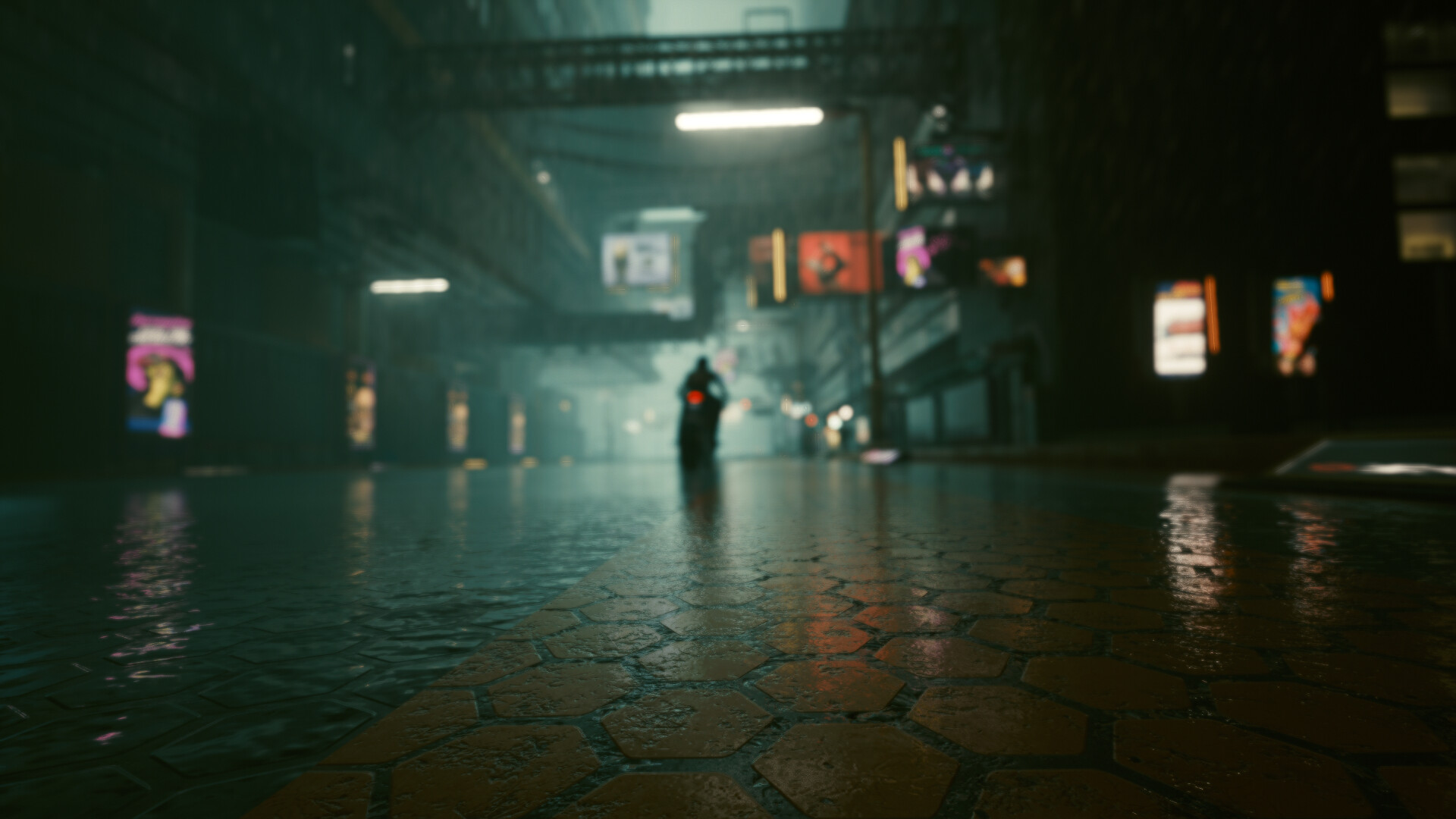The image depicts a rainy night scene from a street-level perspective. Dominating the view is a wet, red-colored stone walkway that immediately transitions to a gray section on the left. The visual is somewhat blurry in the distance, conveying an industrial atmosphere with overhanging lights suspended about two stories up and horizontal scaffolding adding to the utilitarian environment. Crucially, a motorcycle and its rider, rendered as a black silhouette illuminated by a red taillight, are heading away from the viewer, adding a sense of mystery and slight unease.

To the right, a building stands illuminated with vibrant advertisements that resemble television screens, projecting red, yellow, and purple hues. On the left, closer to the viewer, a train bridge crosses overhead, each of its supporting pillars adorned with additional screens showing movie advertisements or other visuals. Elevated steel beams or a possible bridge structure create a canopy overhead between the buildings. Various signs, likely vending or soda machines, populate the streetscape, reinforcing the urban setting.

Amid the dark ambiance, the lighting from the advertisements and street lamps punctuates the scene, highlighting details like cracks in the yellow-lined asphalt. Overall, the staging and imagery evoke the feeling of being within a night-time metropolitan environment, possibly within a video game, characterized by its rich, detailed, and immersive urban landscape.